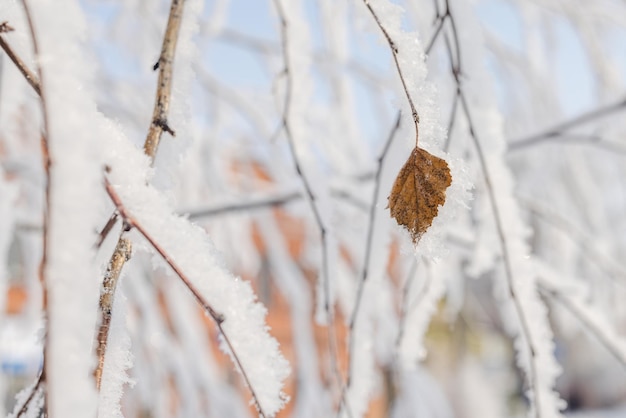This winter photograph, slightly wider than tall, captures a serene and frosty scene centered around a single resilient leaf clinging to a branch. The brown, almost orange leaf with its worn and broken edges stands out against the myriad of snow-covered twigs and branches. The branches vary in size, with the largest being about half an inch in diameter, and a mix of brown and red hues. Snow and frost delicately coat the limbs, emphasizing the coldness of the scene. In the background, a misty tableau with hints of orange elements and blurred green and blue sky create a soft, dreamy contrast to the sharp focus on the leaf and branches. The overall effect highlights the solitary leaf's defiance in the face of winter's grip, complemented by the intricate formations of snow and ice on the surrounding limbs.